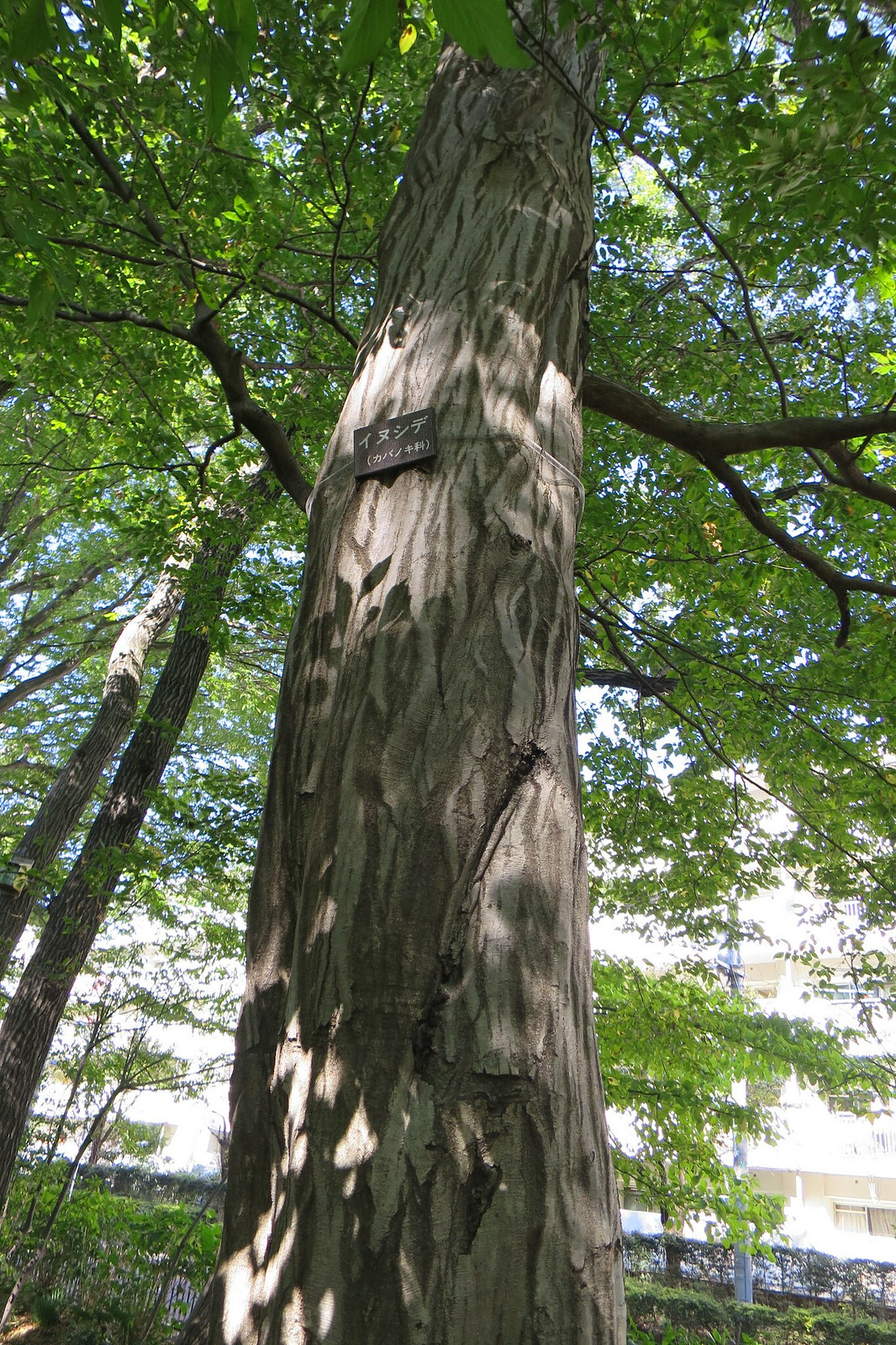In this striking portrait-style photograph, the focus is a towering, majestic tree shot from an upward angle that captures the thick, smooth texture of its bark and emphasizes the impressive height of the trunk. Affixed to the middle of the trunk is a small black sign with white Japanese hiragana characters, labeling the tree. Surrounding this central tree are other smaller, shorter trees, their tops lush and green while their bases reveal more brown. In the background, a black fence encircles the area, leading out to glimpses of city life, including light posts and parked cars, underscoring the tree's urban park setting.